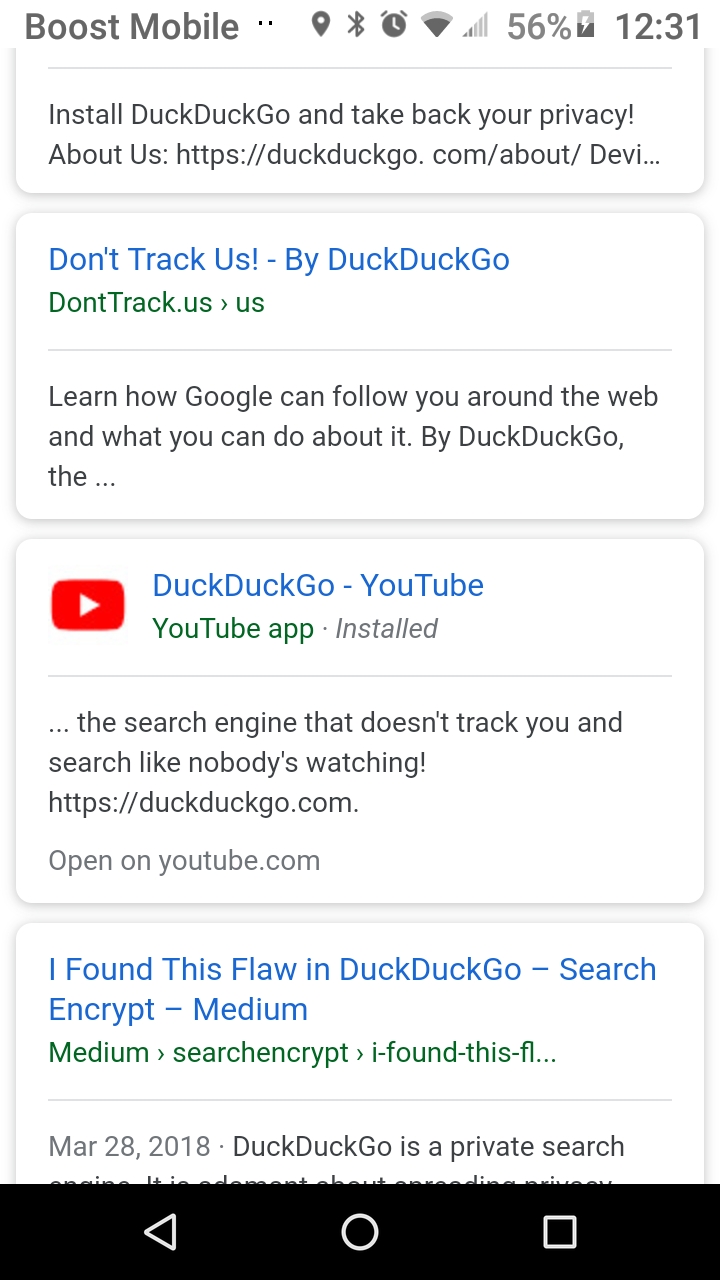In the image, we have a close-up view of a smartphone screen. At the top of the screen, the status bar prominently shows the Boost Mobile carrier. Key indicators include the pin icon, Google or Bluetooth symbol, alarm clock icon, Wi-Fi strength, and battery life at 56%, with a lightning bolt symbol indicating that the phone is currently charging. The time displayed is 12:31.

Below the status bar, several notifications and advertisements can be seen. The first notification is promoting the installation of DuckDuckGo, emphasizing its privacy features. The next advertisement reads "Don't track us by DuckDuckGo" in blue text, followed by a green text line reiterating "Don't track us" in slightly smaller font. Beneath this, in black text, it states, "Learn how Google can follow you around the web and what you can do about it."

Following this, there is a snippet about DuckDuckGo from YouTube, with the description reading, "The search engine doesn't track you, it's like nobody's watching." It provides an option to open the video on YouTube.com.

The final notification is partially cut off but starts with, in blue, "I found this flaw in DuckDuckGo, search encrypt medium," and continues underneath with "medium" followed by a rightward arrow, and "search encrypted" before being cut off. This post is dated March 28, 2018, and mentions DuckDuckGo as a private search engine before getting truncated.

At the bottom of the screen, a black navigation bar features three main buttons: a back arrow on the left, a circular home button in the center, and a square multitasking button on the right.